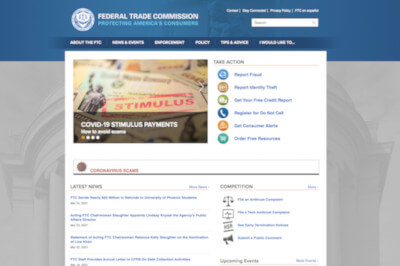This image is a detailed screenshot of the Federal Trade Commission's (FTC) website. At the very top, a blue banner displays the white FTC logo and the text "Federal Trade Commission" in white. Directly beneath this banner, the phrase "Protecting America's Consumers" is prominently featured in blue, though the font may be slightly difficult to read.

To the right, there is a white search box and a series of white navigation submenus. Further down, another set of white submenus is visible, followed by a section titled "COVID-19 Stimulus Payments" in white text. This section includes an image depicting checks with a green background, a Statue of Liberty icon, and the word "STIMULUS" stamped across it in red.

On the right side of this section, there is a series of blue submenus adorned with colored circular icons. Each icon is white, set against a backdrop of various colors including blue, gold, green, dark blue, orange, and teal.

Below this, a prominent red text with a seal beside it is displayed. As we continue scrolling down, there is a "Latest News" section in black text, accompanied by several clickable blue links. Opposite this section, black font text is interspersed with blue words and various icons, including the scales of justice, a gavel, and a bullhorn.

At the very bottom of the image, more text can be seen in black and blue font, completing the comprehensive layout of the FTC webpage screenshot.